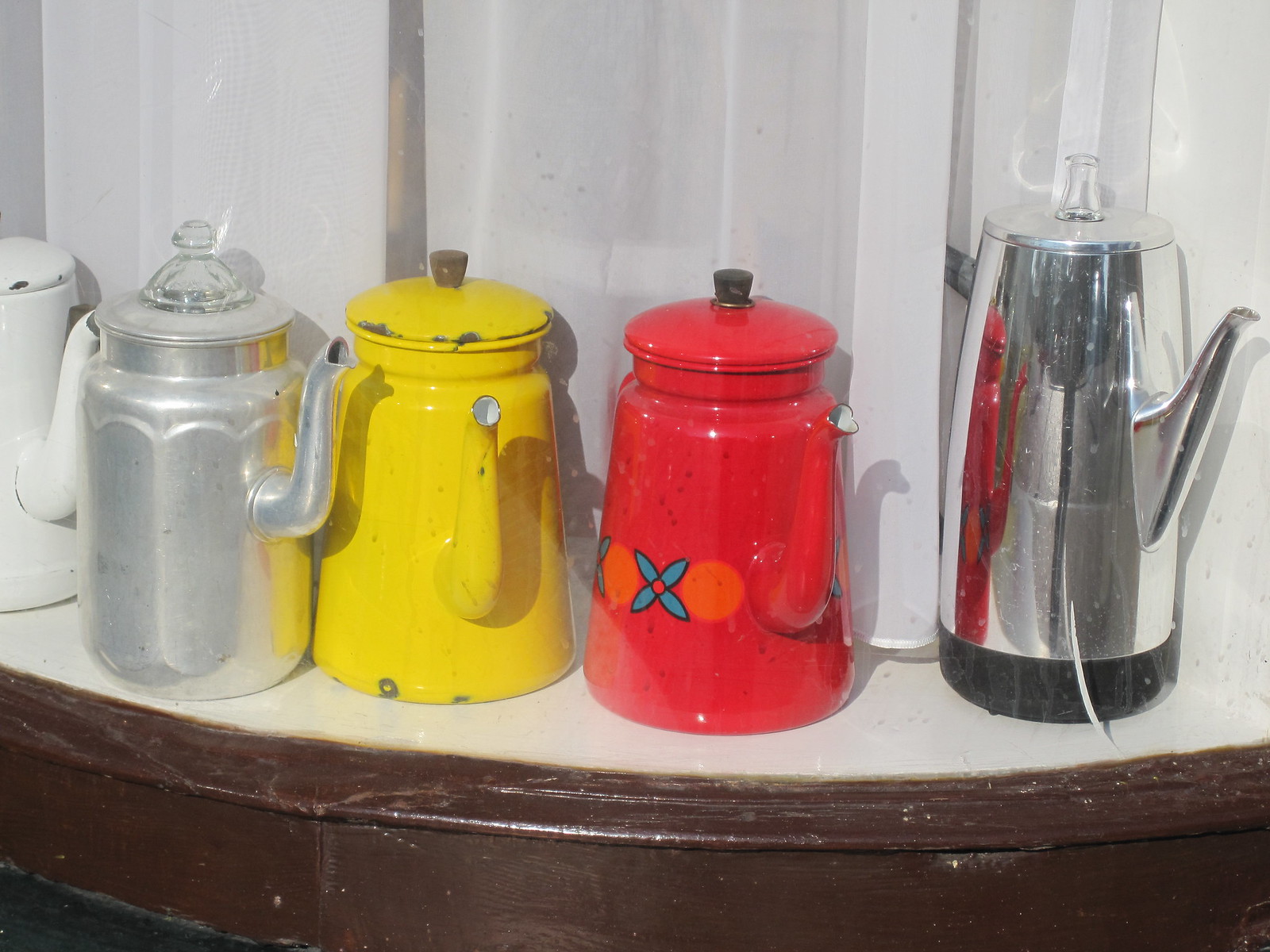This detailed color photo, taken indoors, captures a dark brown shelf or countertop positioned against a wall with white curtains in the background. Arranged neatly on this shelf are five unique teapots, each of different styles and materials. Starting from the left, the first teapot is white ceramic, followed by a grayish tin or aluminum pot with a glass lid. Next is a cheerful yellow ceramic teapot, and to its right is a vibrant red teapot adorned with a distinctive blue flower and two orange circles. The next teapot is tin or stainless steel, reflecting the red teapot beside it. The final item on the right is a tall, modern, stainless steel electric tea kettle with a glass lid. The symmetrical arrangement and variety of colors and materials of the teapots create an eye-catching display against the backdrop.